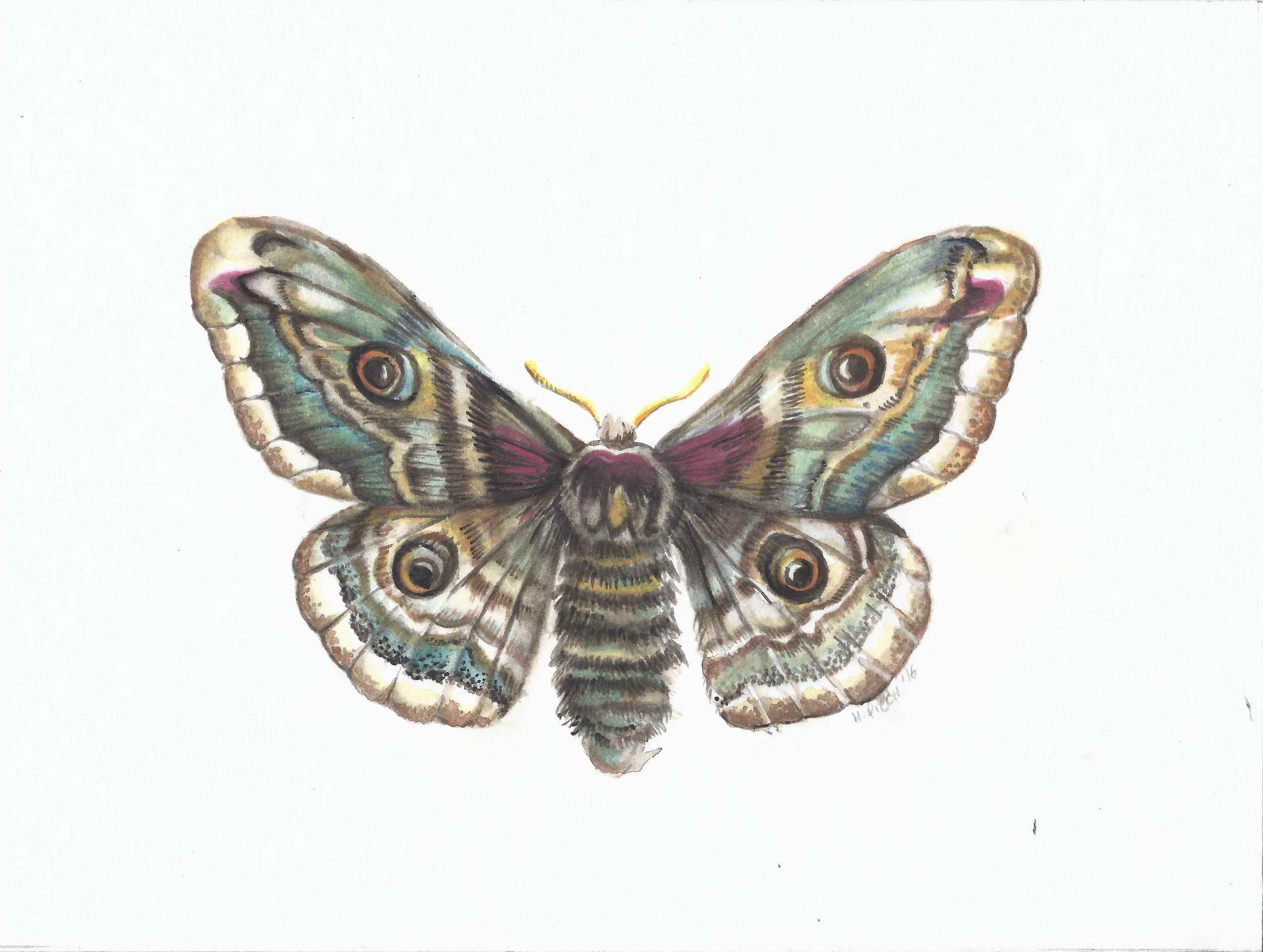This image features a highly detailed and colorful drawing of a moth, set against a white background. The moth’s most striking feature is its ornate wings, which are adorned with patterns that include four eyespot shapes—one on each quadrant of the wings. These eyespots sit amid a vibrant array of colors: there are dominant hues of light blue, cerulean, teal, and purple, with accents of yellow and brown. The edges of the wings display a distinctive brown border, while closer to the body, the hues transition to reddish tones.

The moth's furry, striped body includes black, white, blue, and yellow stripes, adding to the intricate detail of the drawing. The head of the moth features pronounced yellow antennae and a purple triangular or bowtie-shaped marking.

Overall, the rich and varied palette, combined with the detailed textures of the wings and body, suggest that this could be an illustration from a specialized textbook, possibly depicting a rare or exotic species.